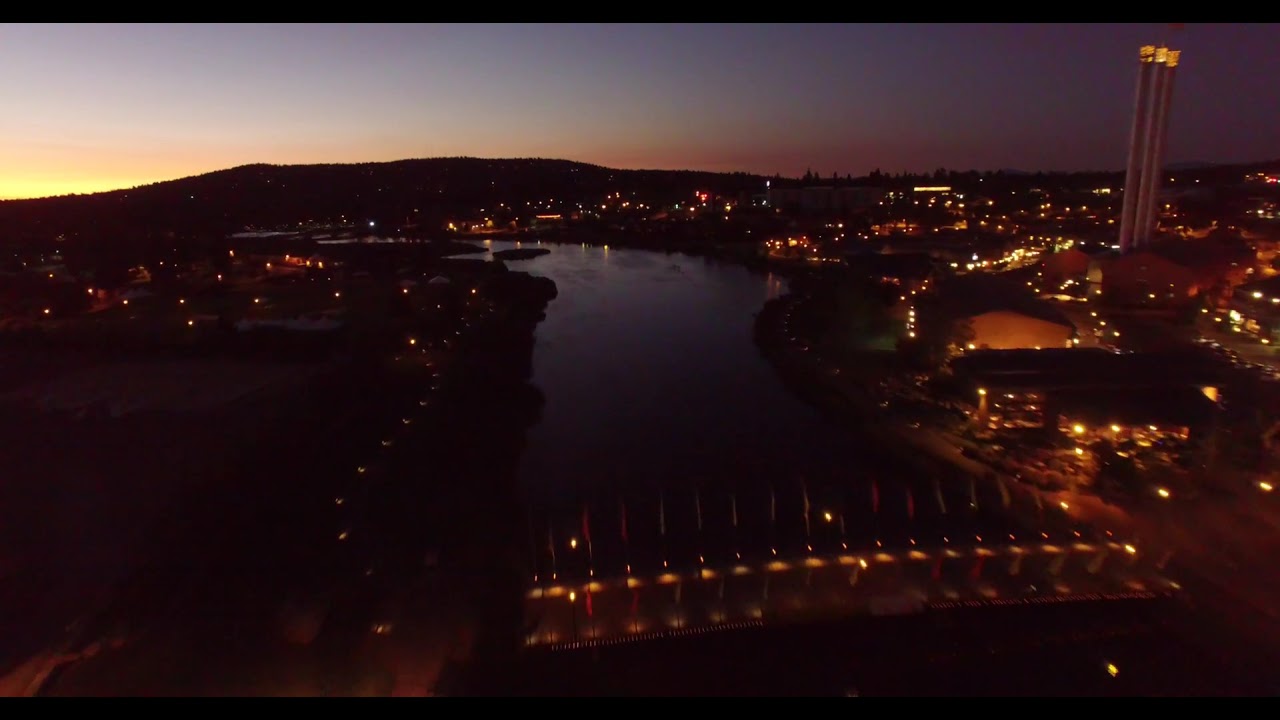This image captures an evening or possibly night-time urban landscape as the sun sets—or has recently set—in the backdrop. The central focus is a river that extends from the foreground to the horizon, appearing almost black save for a sliver of light reflecting off its center. Spanning the river is a bridge illuminated with yellow lights in segmented intervals. To the right, a vibrant cityscape glows with various yellow lights, highlighted by a towering white structure with three columnar sections capped by orange lights. Distant, silhouetted hills form a dark horizon against a gradient sky that transitions from light yellow on the left to deep, dark purple on the right, indicating the fading presence of the sun.